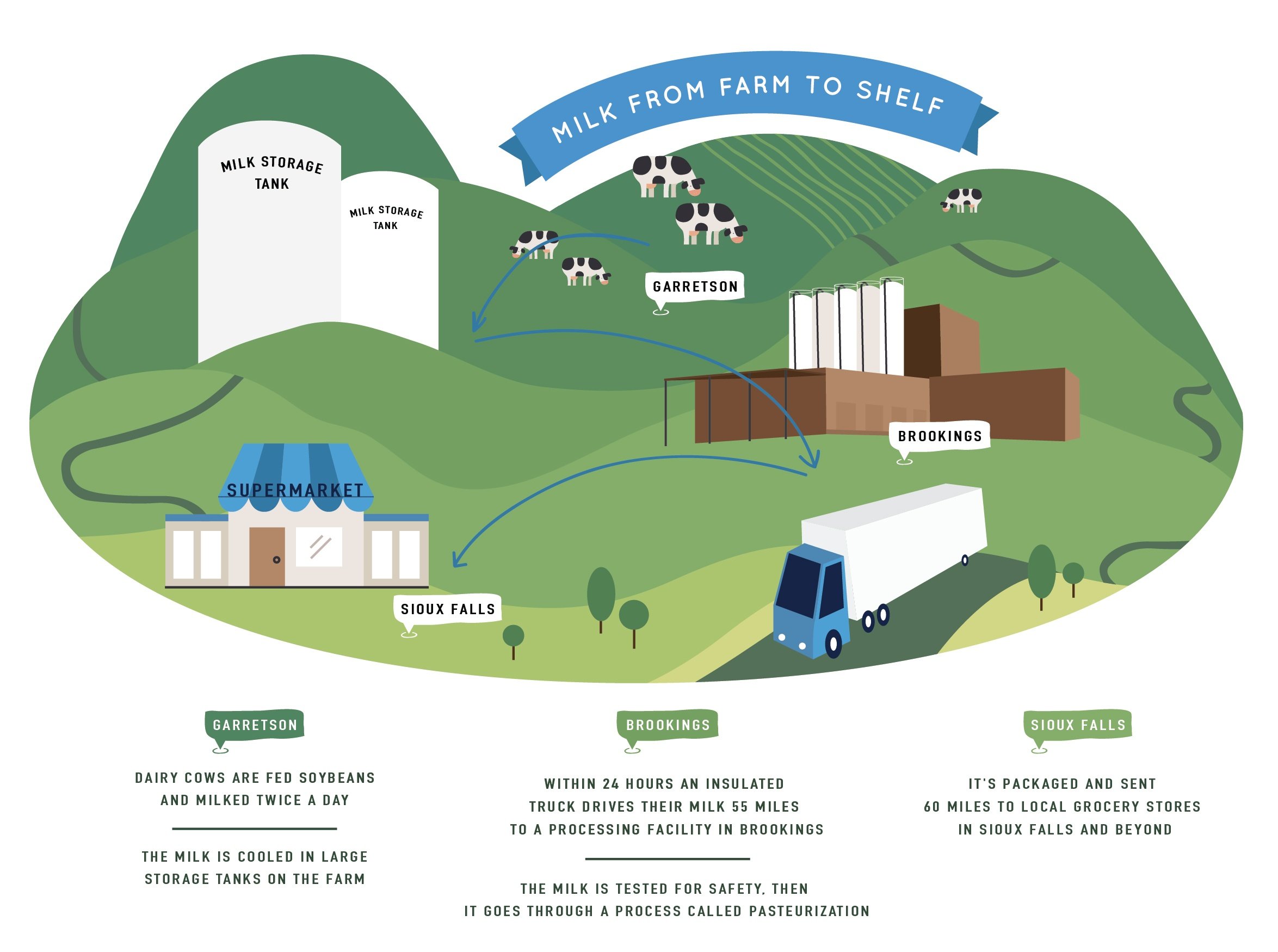The image is a detailed flow chart illustration titled "Milk from Farm to Shelf." It visually depicts the journey of milk from dairy farms to supermarket shelves with a series of drawings and text labels. 

The top caption reads "Milk from Farm to Shelf." The flow chart begins with cows grazing on green hills in an area labeled Garretson. These dairy cows are fed soybeans and milked twice a day. Their milk is initially cooled and stored in large milk storage tanks on the farm. To the left, a set of tanks is specifically labeled "milk storage tanks."

Next, the illustration shows a brown building with five cylindrical structures, signifying a processing facility in Brookings. Within 24 hours, the milk is transported in an insulated truck 55 miles to this processing facility. Here, the milk is tested for safety and goes through a process called pasteurization.

From Brookings, the milk is then packaged and loaded onto a tractor trailer with a blue cab and a white trailer. This truck travels down a depicted road to deliver the milk to a supermarket. The supermarket, prominently labeled "supermarket," is located in Sioux Falls, 60 miles away. The caption notes that the milk is sent to local grocery stores in Sioux Falls and beyond.

In summary, the image details the process of how milk moves from Garretson farms to a Brookings processing facility, and then to supermarkets in Sioux Falls, explaining each stage comprehensively.